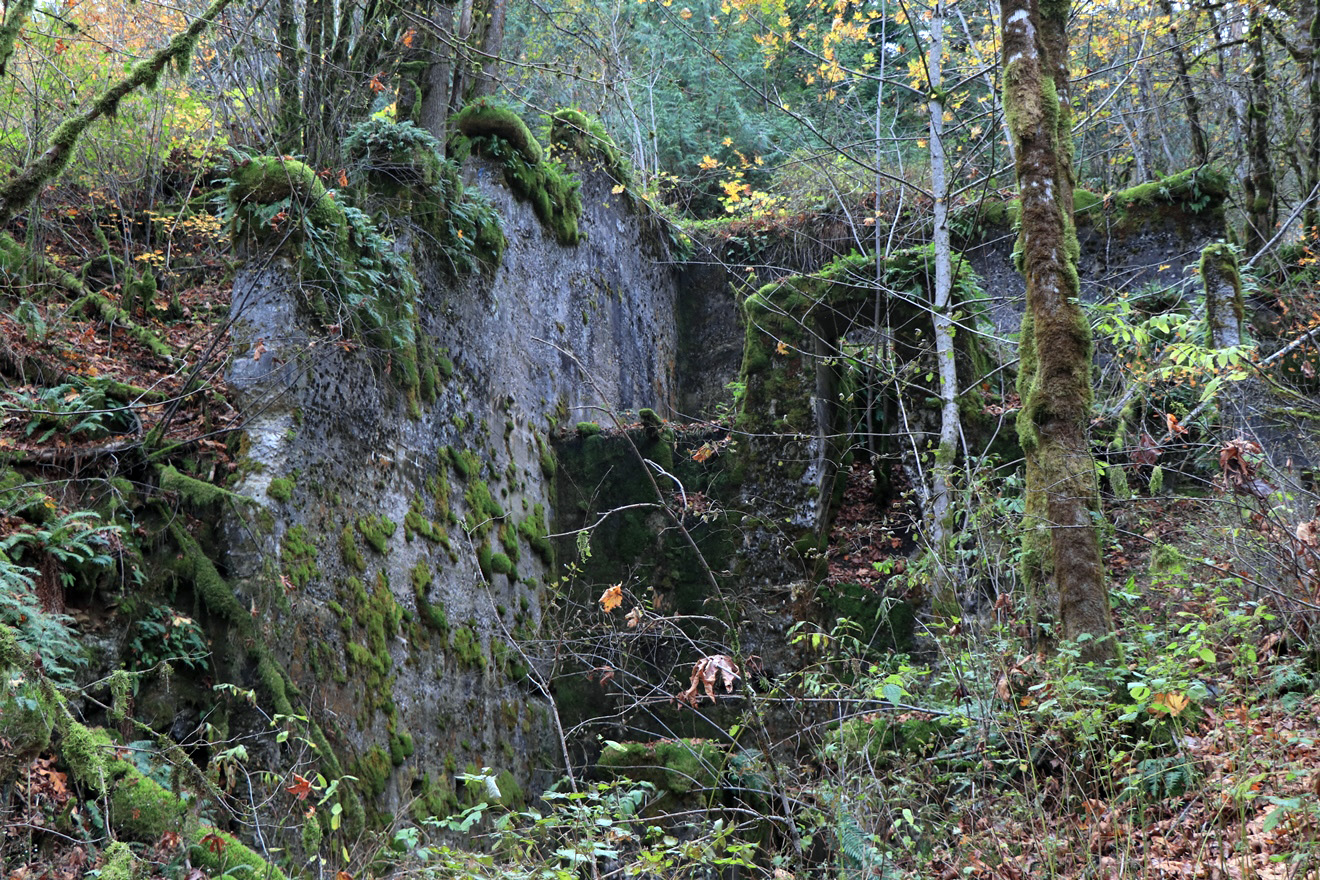The image depicts a heavily overgrown, forested area dominated by the ruins of an old, deteriorated stone or concrete building. Only two walls of the structure remain standing, one of which is heavily covered with green moss, especially concentrated at the top. The remnants suggest it once had stairs, now largely obscured and softened by thick moss. This building appears embedded into a hillside, with a cliff above showcasing numerous deciduous trees adorned with a mix of yellow and green leaves, hinting at a fall season. Additionally, the bottom right corner of the image features a tree trunk extending upward, also blanketed in moss, amidst a forest floor covered with fallen leaves in hues of orange. The scene evokes a sense of abandonment and natural reclamation, reminiscent of something from a 'Jurassic Park' setting, and portrays a lush, verdant environment likely found on the West Coast.